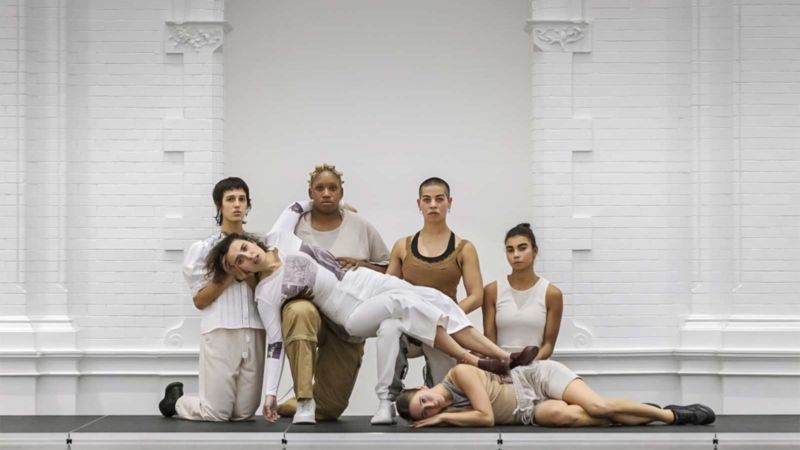The image depicts a group of six drama students, likely on a stage, against a background that combines white brick and decorative white smooth panels. They are dressed in light-colored clothing, primarily whites and sandy browns, with black or white shoes. The group arrangement is notably expressive: 

- In the foreground, a woman is lying down on the floor, facing the camera with her hands positioned behind her head.
- To her immediate left, another woman is seated normally, looking contemplative.
- Further left, two women are kneeling with one knee propped up.
- A central figure, a woman in white with brown-black hair, appears to be lying supine across the laps of these two kneeling women, looking visibly upset or lost in thought. Her legs rest on the lap of the woman on the floor, and her head is slightly supported by the woman kneeling at the far left, who is also on both knees.

The backdrop includes artistic columns and a white-brick design with smoother, decorated segments, enhancing the stage's theatrical ambiance. The black mat beneath them further suggests they are performing or rehearsing a scene. Overall, the scene is laden with emotion, as indicated by the solemn expressions and intricate posing of the students.